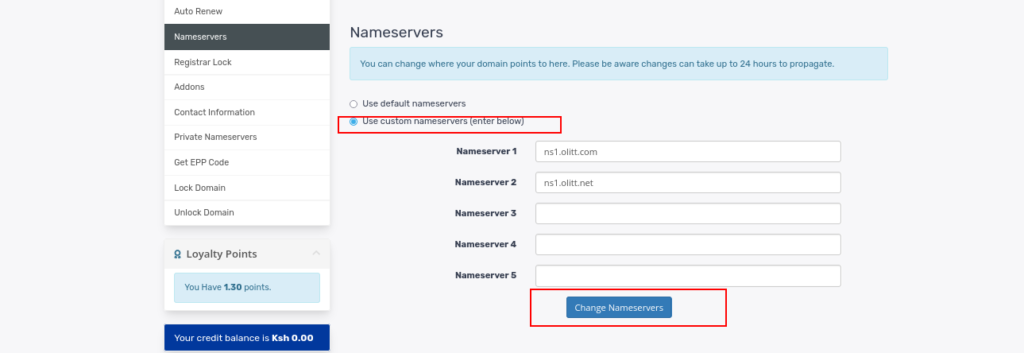The image is a screenshot of a web management interface, displaying various settings related to domain management. 

The background is primarily gray with distinct sections in white, blue, and black. Key areas are highlighted with a red rectangle, providing emphasis. At the top of the screenshot, the menu begins with "Auto Renew" and continues vertically listing options such as "Name Servers," "Register Lock," "Add-ons," "Contact Information," "Private Name Servers," "Get EPP Code," "Lock Domain," and "Unlock Domain." The "Name Servers" section is currently active and expanded.

In the detailed "Name Servers" section, a blue dialog box contains text that explains, "You can change where your domain points to here. Please be aware changes can take up to 24 hours to propagate." A specific subsection titled "Use custom name servers, enter below" and a prompt labeled "Change name servers" are both enclosed within a red rectangle, indicating their importance. Additionally, the user's loyalty points are visible, showing they have "1.30 points," along with a credit balance of "KSH 0.00."

A blue dot next to the option indicates it's selected, signifying an active choice in the process of managing or altering the domain’s name servers.